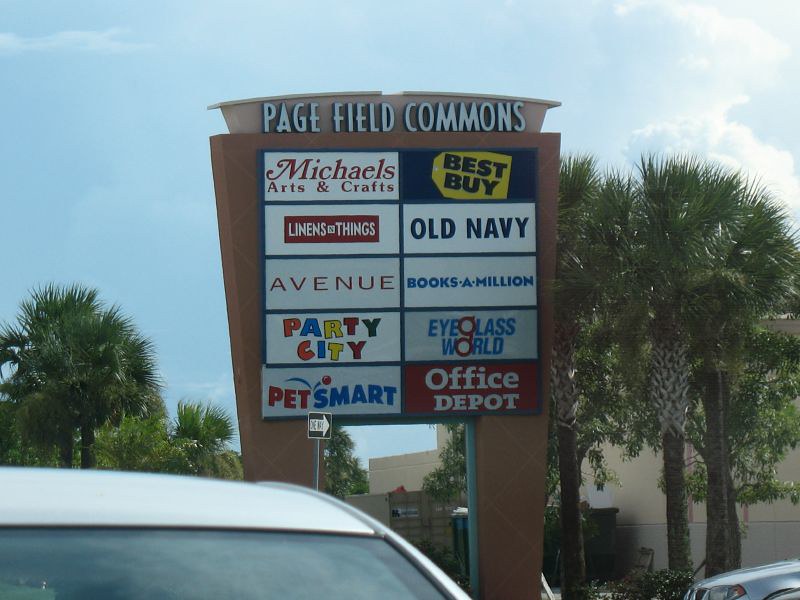This image depicts a large, structured sign located at the entrance of a shopping mall named Page Field Commons. The sign prominently displays a list of the mall's prominent retailers, each separated into distinct segments. The businesses listed from top to bottom are Michael's Arts and Crafts, Linens and Things, Avenue, Party City, PetSmart on the left side, and Best Buy, Old Navy, Books a Million, Eyeglass World, and Office Depot on the right side. The foundation of the sign is constructed from a dark red clay material, adding a robust and organic touch to its design. In the background, tall palm trees sway gently, adding a touch of tropical ambiance, while the hood of a nearby car peeks into the frame from the bottom. This detailed sign serves as an inviting gateway to the various shopping experiences that Page Field Commons has to offer.